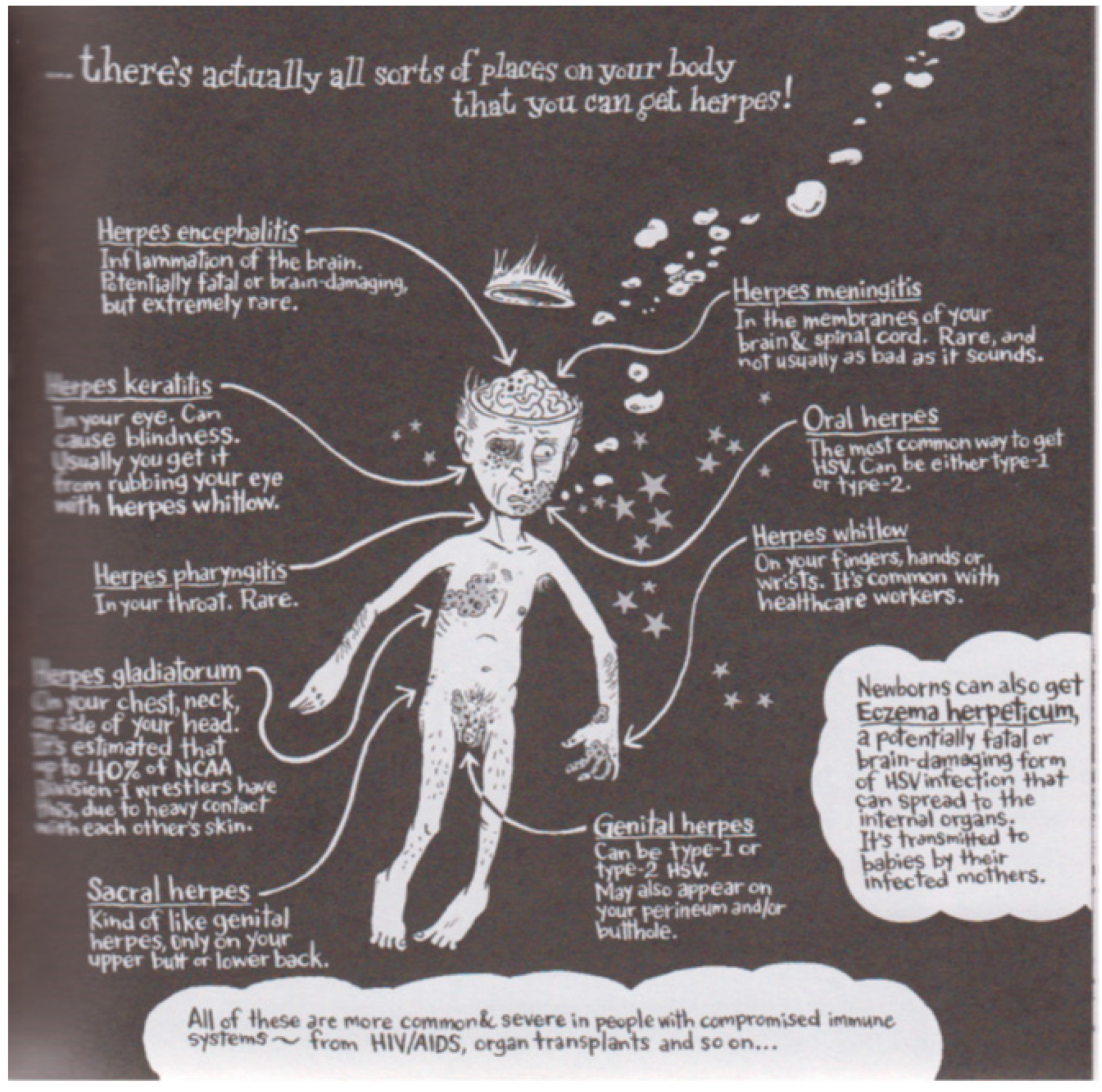The infographic image, which appears to be a cutout from a magazine, illustrates a herpes awareness campaign against a dark gray or black background. At the center of the image is a cartoonish, floating naked man with a dazed and confused expression. His scalp is removed, exposing his brain, and the detached part of his head hovers above like a crown. Around the man, white arrows point to various parts of his body, highlighting different places where herpes can occur. The text at the top of the image states, "There are actually all sorts of places on your body that you can get herpes." Additional white text details various types of herpes and their effects, including information about neonatal herpes and the severity of the disease in those with compromised immune systems. White text bubbles are scattered around the image, with more concentrated paragraphs at the bottom, depicting general information about the disease, all set against the stark black background which enhances the eerie, somewhat creepy atmosphere of the diagram.